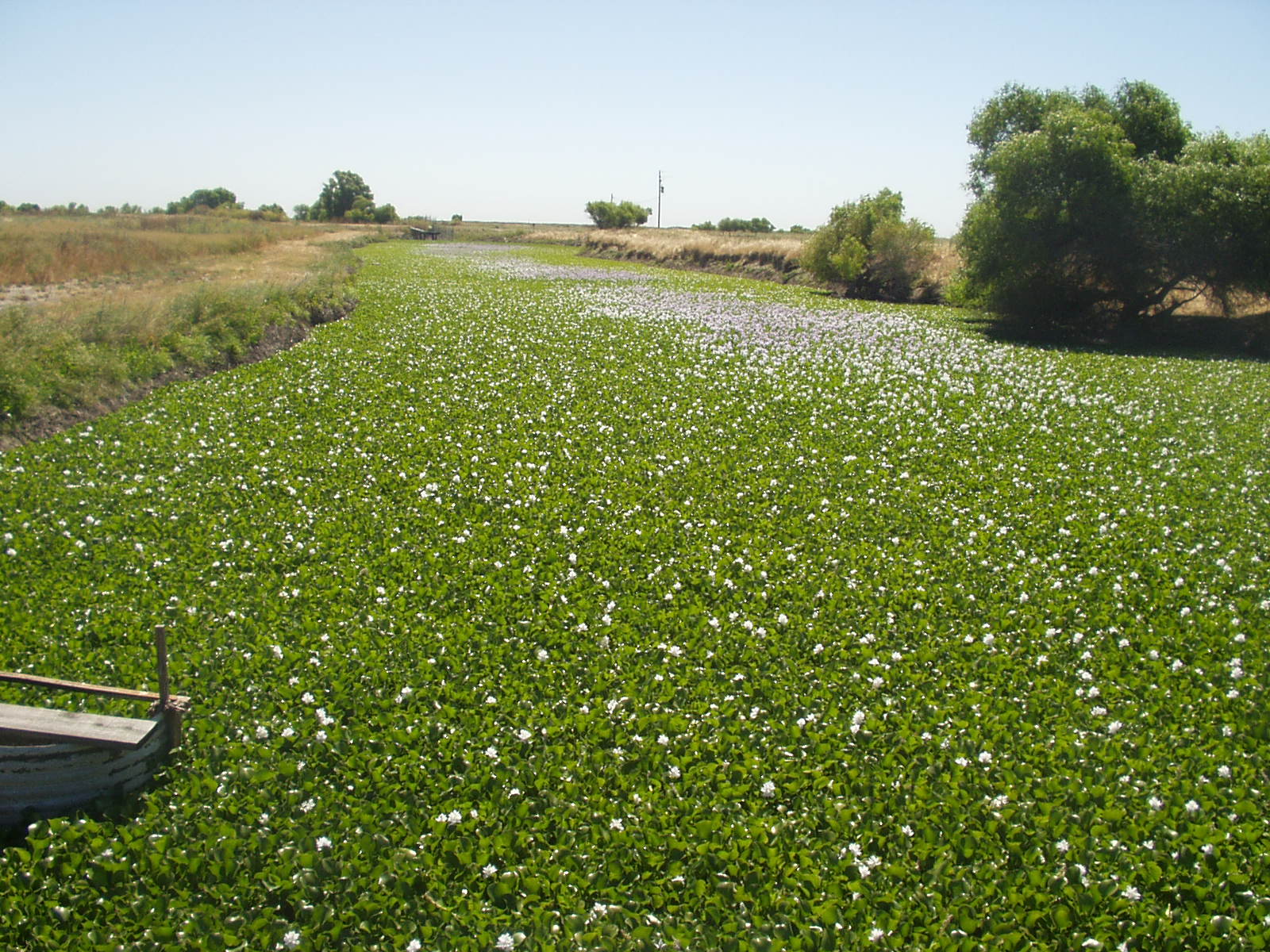This daytime photograph showcases a sunlit field under a clear, cloudless blue sky. The field is carpeted with lush greenery and sprinkled with white flowers, which become denser towards the middle distance of the image, resembling a meandering river of blossoms. The visual effect is such that what appears like a winding waterway is actually a vibrant flowerbed cutting through the field. To the bottom left, a small brown wooden object rests on the land, near a slight rise in the ground. Tall trees border the scene on both sides, along with a solitary telephone pole visible in the distance. Scattered throughout the expanse of land are patches of hay or weedy growth, adding texture to the field's surface. In the immediate background, more large, leafy trees frame the picturesque landscape.